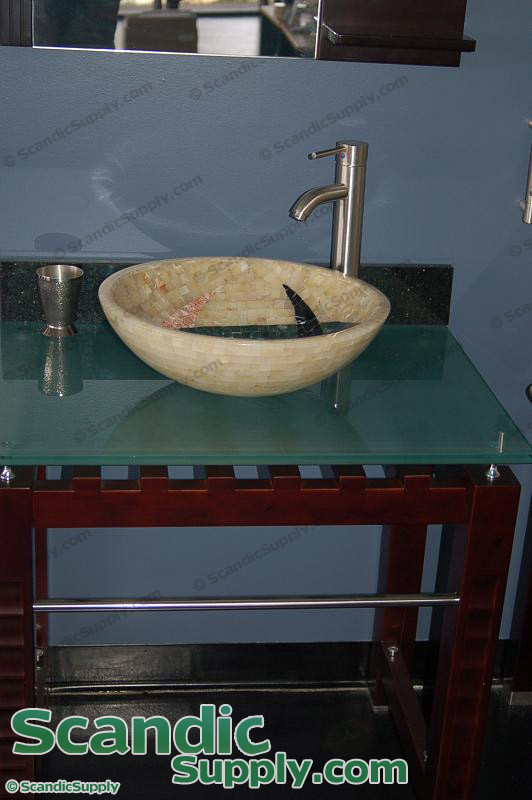This promotional image for ScandicSupply.com showcases an elegant bathroom vanity setup. The centerpiece is a sophisticated modern sink, featuring a sleek bowl design. The bowl itself is a striking combination of beige with subtle light red accents, creating a visually appealing effect. A stylish silver faucet elegantly arches above the bowl, adding to the modern aesthetic.

The sink is supported by a light blue glass table, which rests on a compact, brown wooden cabinet. The cabinet integrates seamlessly with the glass table, which is secured by a horizontal silver bar connecting its legs. Next to the sink, a small silver jigger-like accessory adds a touch of detail and functionality.

In the background, the Scandic Supply Company logo is prominently displayed on the wall, indicating the brand behind this contemporary and chic bathroom ensemble.